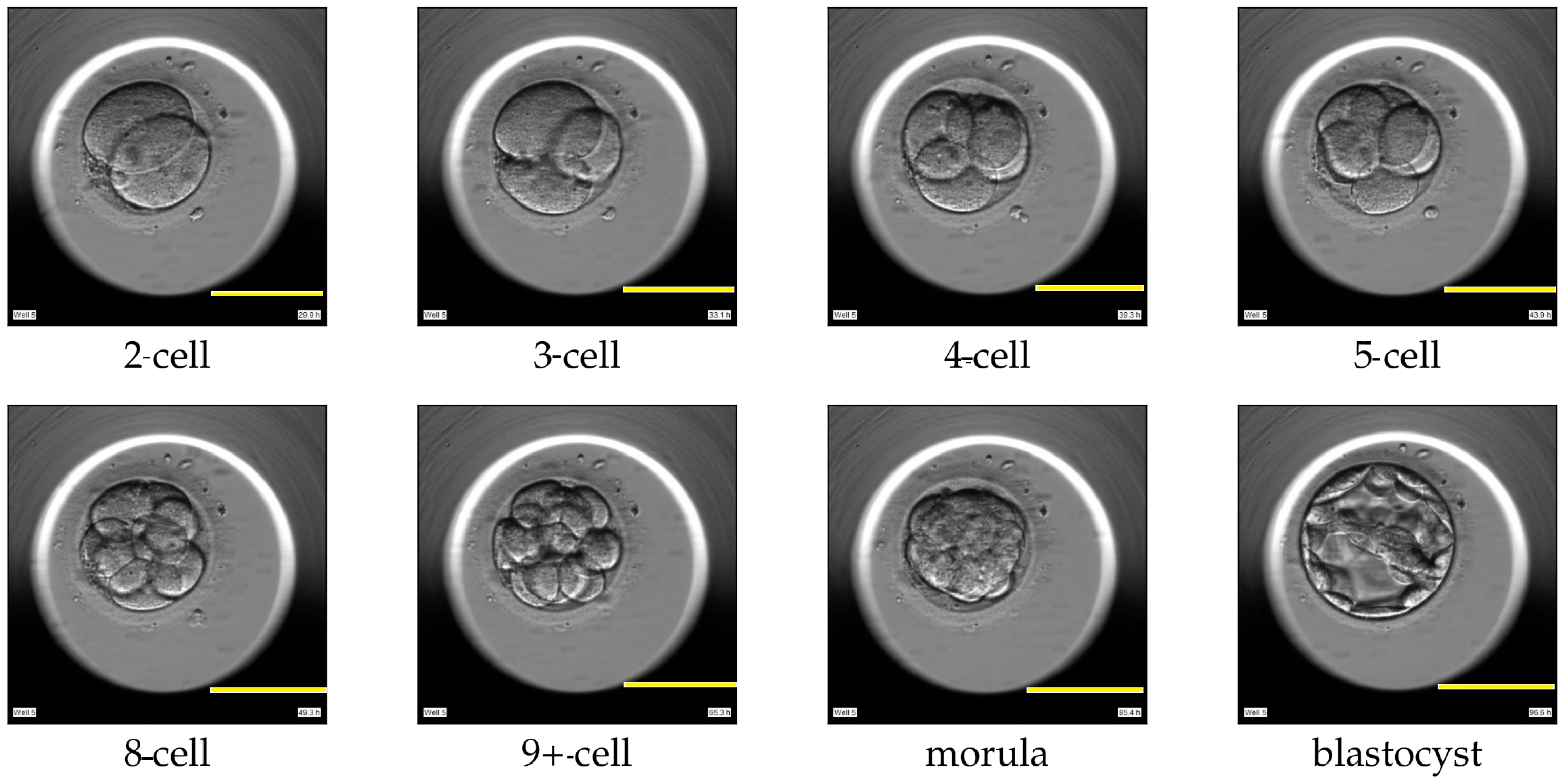The image appears to be an educational diagram, likely from a science textbook, showcasing the stages of early embryonic development. It features eight small, square diagrams arranged in two rows of four, each with a gray background. The diagrams resemble small silver batteries with intricate designs that include multiple interconnected circles.

In the top row, from left to right, each square is labeled beneath with the corresponding number of cells depicted in the center of the circles: "2 cell," "3 cell," "4 cell," and "5 cell." Each designation is accompanied by a visual representation of the respective cell number.

Similarly, in the bottom row, the squares are labeled: "8 cell," "9+ cell," "morula," and "blastocyst," with the illustrations reflecting these developmental stages. A distinctive yellow line runs to the right of each circular design in every square, further highlighting the specific stage of cellular development.